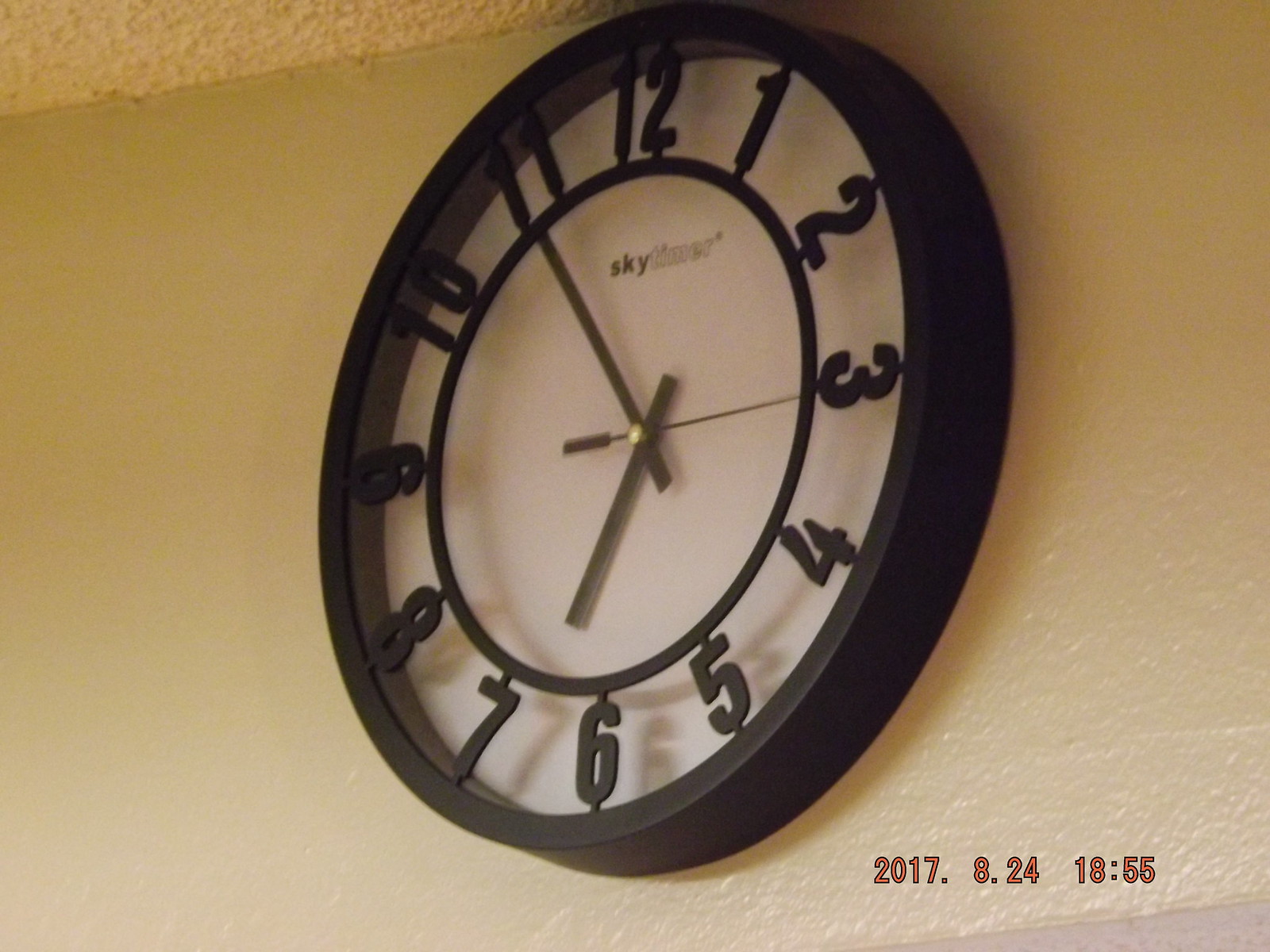This detailed photograph captures a modern circular clock prominently hung on a beige textured wall, with the top portion of the clock nearly touching a white popcorn ceiling visible in the top left corner. The clock features a thick black outer frame and a sleek white face. The black metal numbers (1 through 12) are uniquely connected to both the central black ring and the outer frame, creating an airy, open design without a glass cover. In the center of the clock, the words "Sky Timer" are visible. The clock’s hands, including the hour, minute, and second hands, are elegantly designed in gold. The time displayed on the clock is 6:55, which corresponds to the date and time stamp in red text located at the bottom right corner of the image, reading 2017.8.24 at 1855.